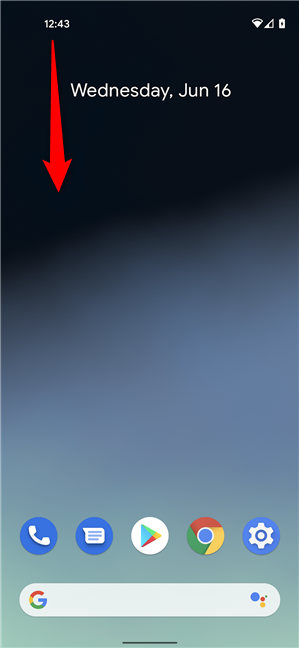The screenshot displays the home screen of an Android mobile device. At the top left corner, the device time is shown as 12:43. Positioned at the top right are three status icons: the Wi-Fi icon, the network signal icon, and the battery icon, indicating that the battery is currently charging. A red or deep orange arrow points downward from the time display, and to the right of this arrow, the date is clearly visible as Wednesday, June 16th.

Below the date, several essential apps are displayed, including the Dialer app, Message app, Google Play Store, Google Chrome, and the Settings app. Further down, the Google Search widget is prominently placed, providing quick access to search functions. Finally, at the bottom of the screen, the navigation buttons are visible for easy navigation.

The home screen wallpaper features a gradient transition that blends from black at the top through blue, culminating in green at the bottom, offering a visually appealing background.